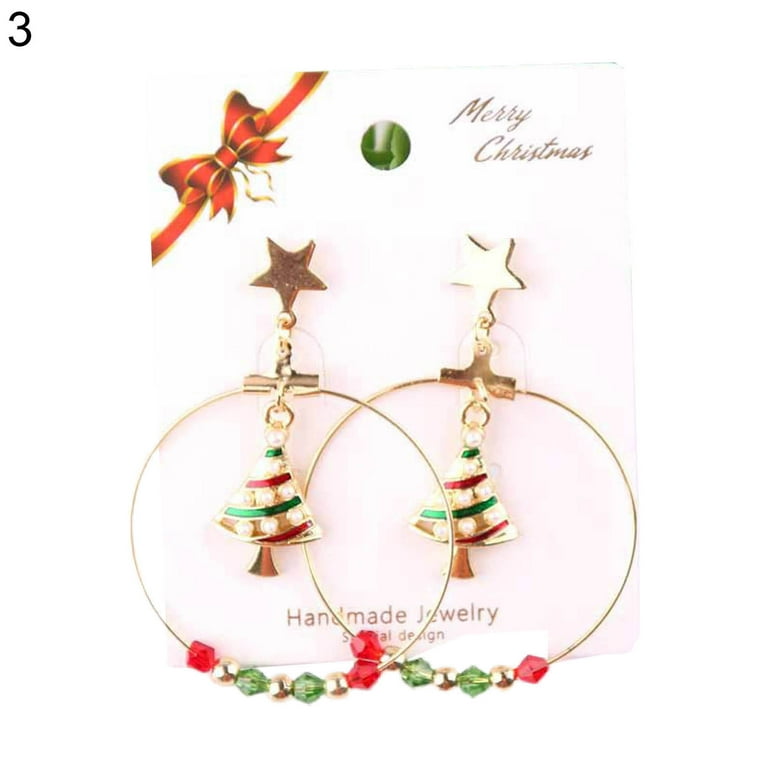This is a color photograph intended for a shopping website showcasing a pair of Christmas-themed handmade earrings. The earrings are attached to their original packaging, a plastic card adorned with festive elements. At the top right corner of the card, "Merry Christmas" is inscribed in gold cursive, while the bottom of the card features the text "Handmade Jewelry" with additional design branding.

The earrings themselves are intricate and festive. Each earring consists of a gold star stud at the top, which serves as the attachment point to the ear. Dangling from the star is a large gold hoop adorned with alternating red and green beads separated by gold balls. In the center of each hoop, a golden Christmas tree with red and green garland, tiny diamond-like ornaments, and a topper star dangles elegantly.

Additional decorative elements include a red bow with gold trim positioned in the upper left corner of the card, emphasizing the holiday theme. The entire setup is displayed against a completely white background with a faint number three in the top-left of the image, suggesting its use in a series for web design or catalog purposes.